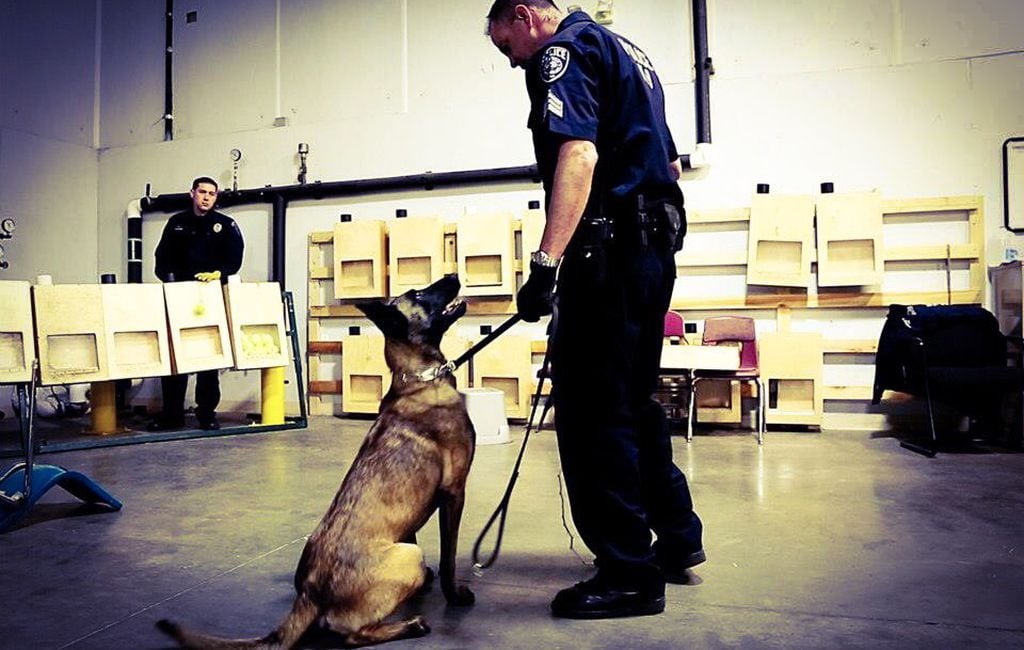In a spacious, indoor setting with a white back wall and a concrete floor, this realistic horizontal photograph captures a moment between a police officer and a German Shepherd. The officer, a white man with short hair, is dressed in a navy blue shirt, black pants, and black gloves, firmly holding the dog's leash with his left hand. The officer is gazing down at the obedient dog, while the dog, sitting attentively, looks up at him. The German Shepherd, a large, dark gray canine with a black face and ears, appears well-trained and alert. Positioned slightly to the left in the background, another police officer with short black hair, wearing a black uniform, watches the interaction. The setting, possibly a warehouse or large storage room, features stacked wood pallets, desks, and chairs against the far wall. There are also visible pipes and gauges along the wall, adding to the industrial feel of the space. The room is neatly organized, with the scene exuding a calm and controlled atmosphere.